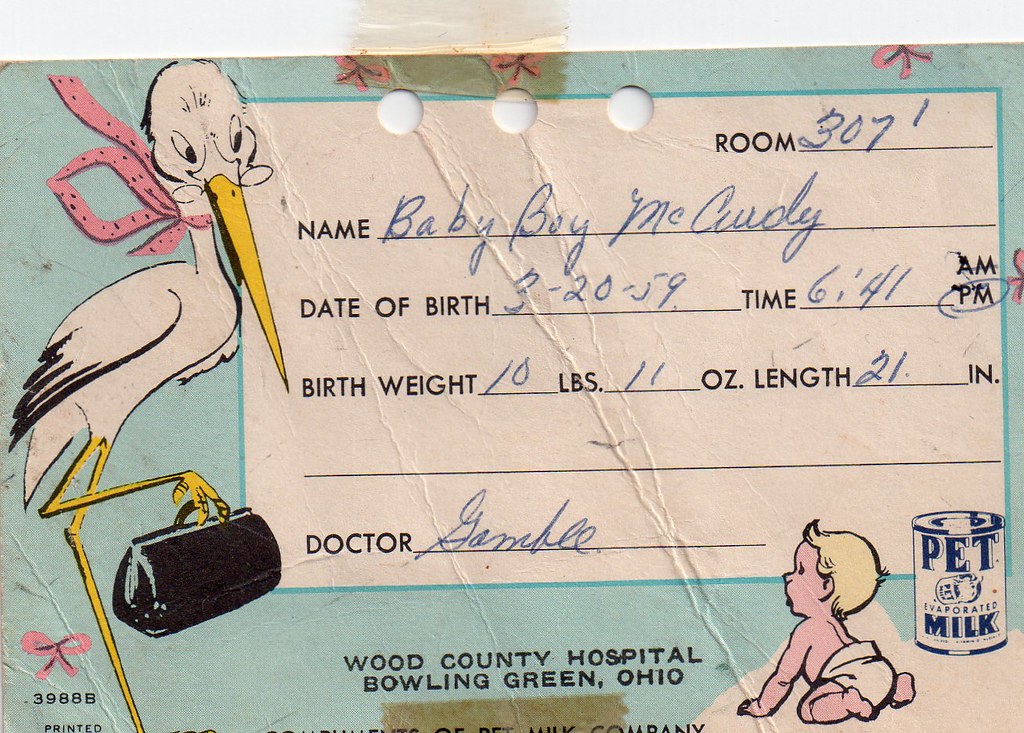This image depicts an old and worn-out birth certificate, filled out with detailed information. It states that the birth took place in Room 307 at Wood County Hospital, Bowling Green, Ohio. The baby boy, named Mick Cuddy or possibly McCurdy, was born on March 20, 1959, at 6:41 PM, weighing 10 pounds and 11 ounces and measuring 21 inches in length. The attending physician is listed as Dr. Gamble. The certificate is very colorful and features various illustrations: on the left side, a large white stork wearing glasses and a pink scarf around its neck is holding a traditional doctor's bag while looking at the baby. On the bottom right corner, there is a drawing of a blonde-haired baby in a diaper alongside a can of Pet Evaporated Milk. The birth certificate also has a blue background and three small holes at the top, possibly intended for a ring binder.